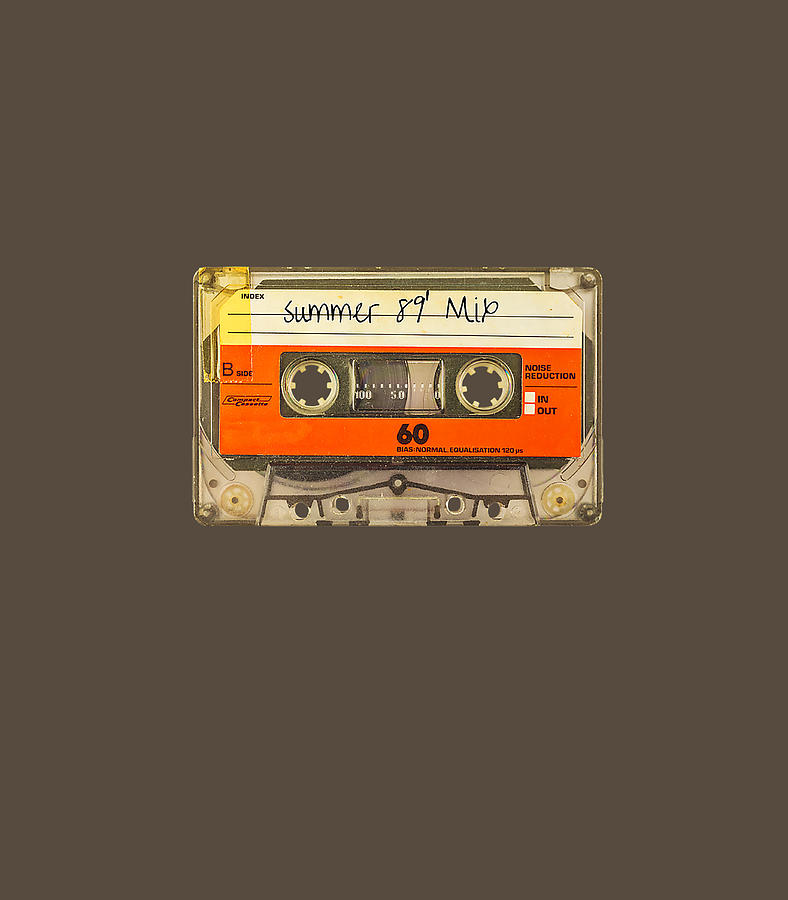This is an image of a detailed drawing, likely digitally altered, of a clear, rectangular cassette tape prominently situated against a dark brownish-gray background. The cassette tape itself showcases a variety of intricate components, such as the internal spokes and several metal screws holding it together. 

The tape features a red and white label. The upper section of the label, which is white, has blue, handwritten text that reads "Summer 89 Mix," indicating it's a mixtape of favorite songs from the summer of 1989. Just below that, the red portion of the label prominently displays "B-side" and the number "60." Additional text on the right side of the tape mentions "Noise Reduction" with checkboxes labeled "in" and "out."

Notably, there is a yellowish piece of tape at the top left corner of the cassette. The drawing captures the old-school vibe of physical media, emphasizing the transparent nature of the cassette, allowing a clear view of the internal mechanisms designed to play the audio tape, further adding to the nostalgia of this classic artifact.